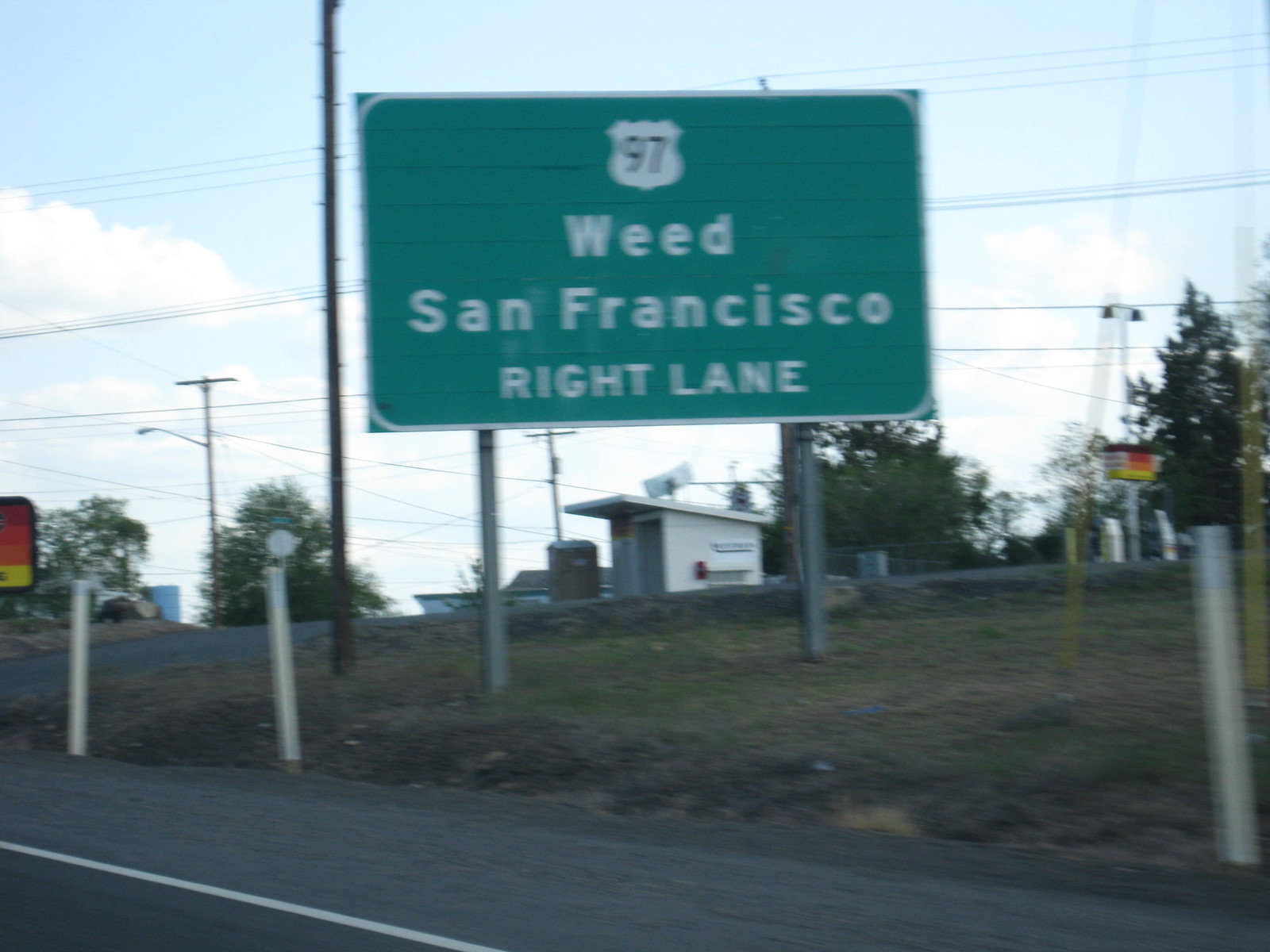The image captures a green highway sign, photographed from a moving car, evident from the motion blur and the partial view of the road along with some guard posts. The sign, located approximately 20-30 feet from the photographer, features a shield symbol with the number "97" inside it. It directs traffic towards Weed and San Francisco, indicating the right lane for the exit. The scene also includes an exit lane veering off to the right. In the background, there are a few trees and a small shed nestled in a dirt lot area, contributing to the rural setting. This humorous snapshot likely caught the photographer's attention due to the amusing juxtaposition of the destinations "Weed" and "San Francisco."